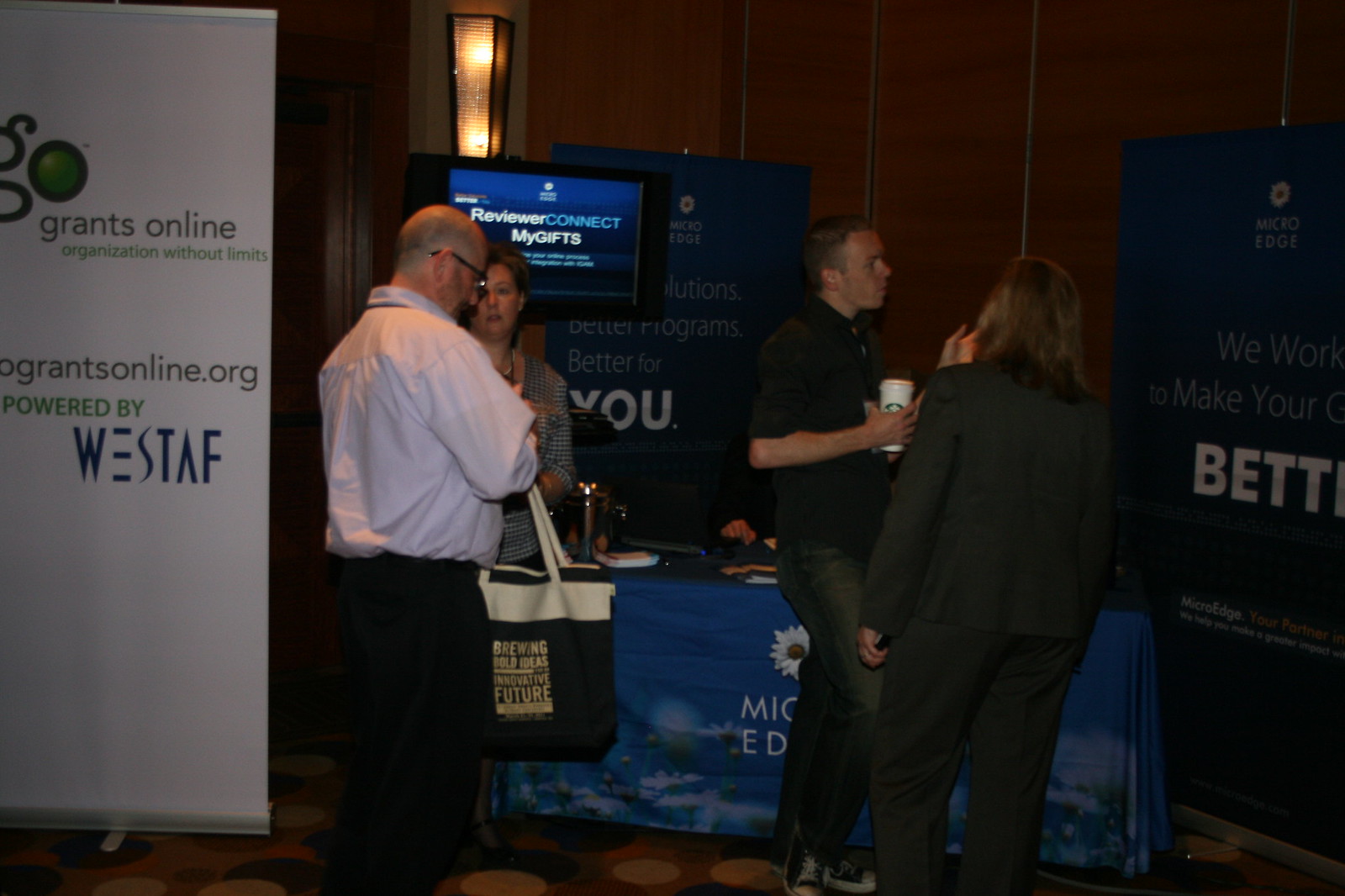The dimly lit image, likely taken at a trade show or convention, captures four individuals congregating around a booth adorned with a blue tablecloth and various marketing materials. The booth, marked by a stand-up white banner, prominently displays the phrases "Grants Online," "Organization Without Limits," and the website "grantsonline.org," powered by WeStaff. On the right, an additional banner features the words "Micro-Edge" and "Reviewer Connect My Gifts" on a TV screen behind them. 

The man in the foreground wears a white button-down shirt, black pants, and glasses, carrying a tote bag. Next to him stands a woman in a checked blouse. To their right, another man dressed in a black polo shirt and jeans holds a Starbucks coffee cup. The fourth person, a woman in a black suit with long brown hair, stands next to him. All appear somewhat disengaged, not looking at each other directly, with one man distracted by his phone. The overall atmosphere is subdued, emphasizing the booth's role as an informational hub for job-seeking services.